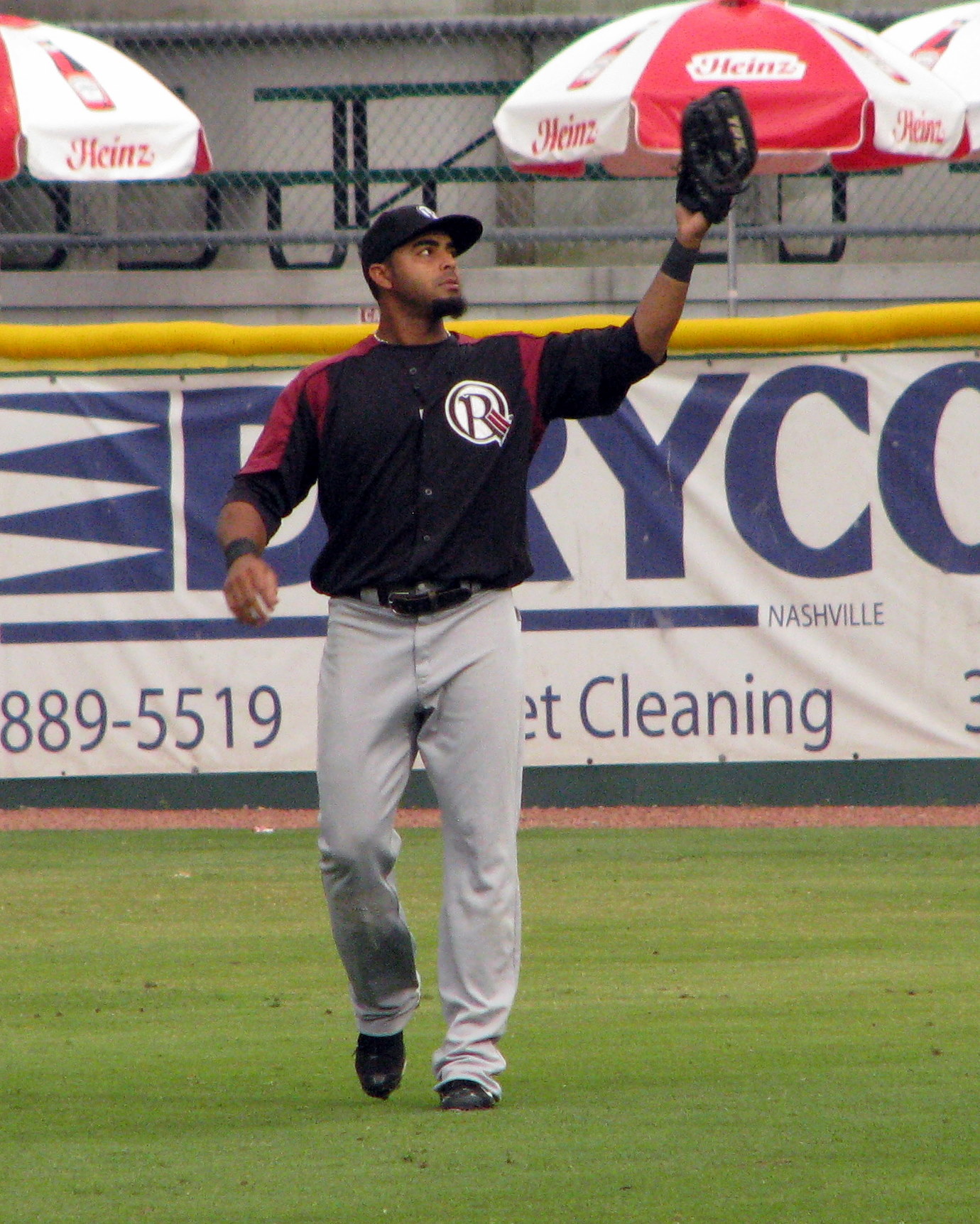The image captures a baseball player standing mid-stride on the green grass of the outfield. He is dressed in light gray baseball pants, black baseball cleats, and a dark blue jersey with burgundy shoulders and sleeves extending to his elbows. The player, who appears to have a short black beard, is looking up into his black glove on his left hand while his right arm, also gloved, is bent at the elbow and slightly extended in front of him. He wears a black or dark blue ball cap featuring white lettering on the front. In the background, a chain-link fence is attached to a concrete wall, partially covered by a white banner that reads "Dryco" and "Nashville," with a partially visible phone number, indicating a potential carpet cleaning advertisement. Red and white patio umbrellas with the Heinz logo and images of ketchup bottles add vibrant accents to the scene.